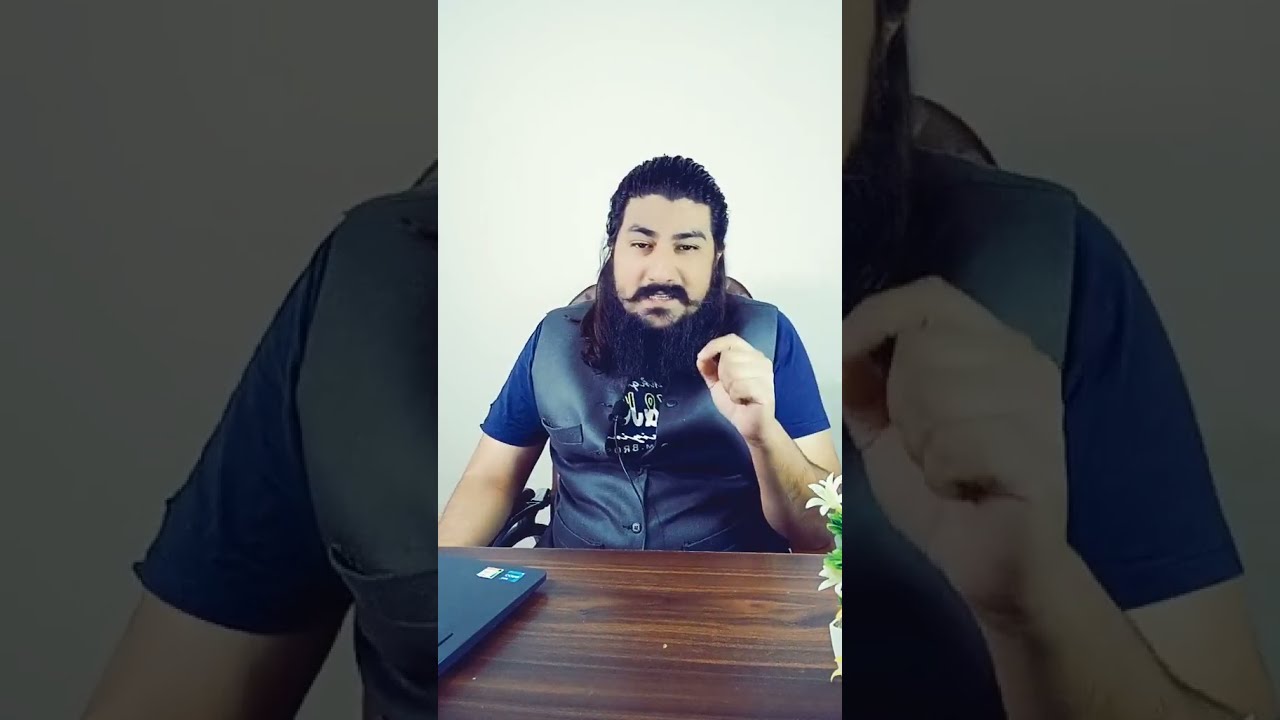A man with short, tight curls of black hair, a handlebar mustache, and a neatly trimmed, bushy black beard sits at a brown wooden table against a plain white background. He has expressive, dark eyebrows and appears to be of Middle Eastern descent, with olive skin. He is wearing a blue t-shirt under a snug black leather vest that has a single button and is equipped with a lapel microphone. The man is gesturing with his left hand, pinching his fingers as if making a point, while his right arm rests down by his side. In front of him, there is a blue book and a small pot with what appears to be an Easter lily or a similar white flower. To his right, though somewhat off-screen, a laptop is visible. He is seated in an office chair, and the setting suggests he might be engaged in a discussion or presentation.